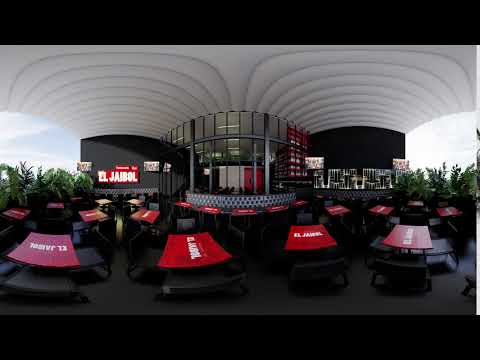The image captures an outdoor seating area of a stylish restaurant, encapsulated within black borders at the top and bottom. Centered in the photo, the restaurant’s white ceiling elegantly arches outward, complemented by black flooring beneath. Dominating the scene are numerous tables with striking red tabletops adorned with white writing that reads "L-J-A-I-B-O-L." 

Flanking both the left and right sides are plants that add a touch of greenery to the sleek setting, while the black walls of the building reinforce the modern aesthetic. The left wall features a red banner with similar white text, contributing to a cohesive color scheme. On the right, outdoor televisions are mounted on the black wall, enhancing the ambiance. 

In the background, a semi-circular counter with stools extends outward, possibly functioning as a bar area, though specifics are obscured. The design elements suggest a high-end dining experience, with large, comfortable seats accompanying the red tables. The overall setting is illuminated by daytime light filtering through clear glass window panes, revealing a sky filled with clouds and an open-air feel on both sides. The photograph's meticulous details and panoramic nature offer a comprehensive view of the trendy, sophisticated restaurant.